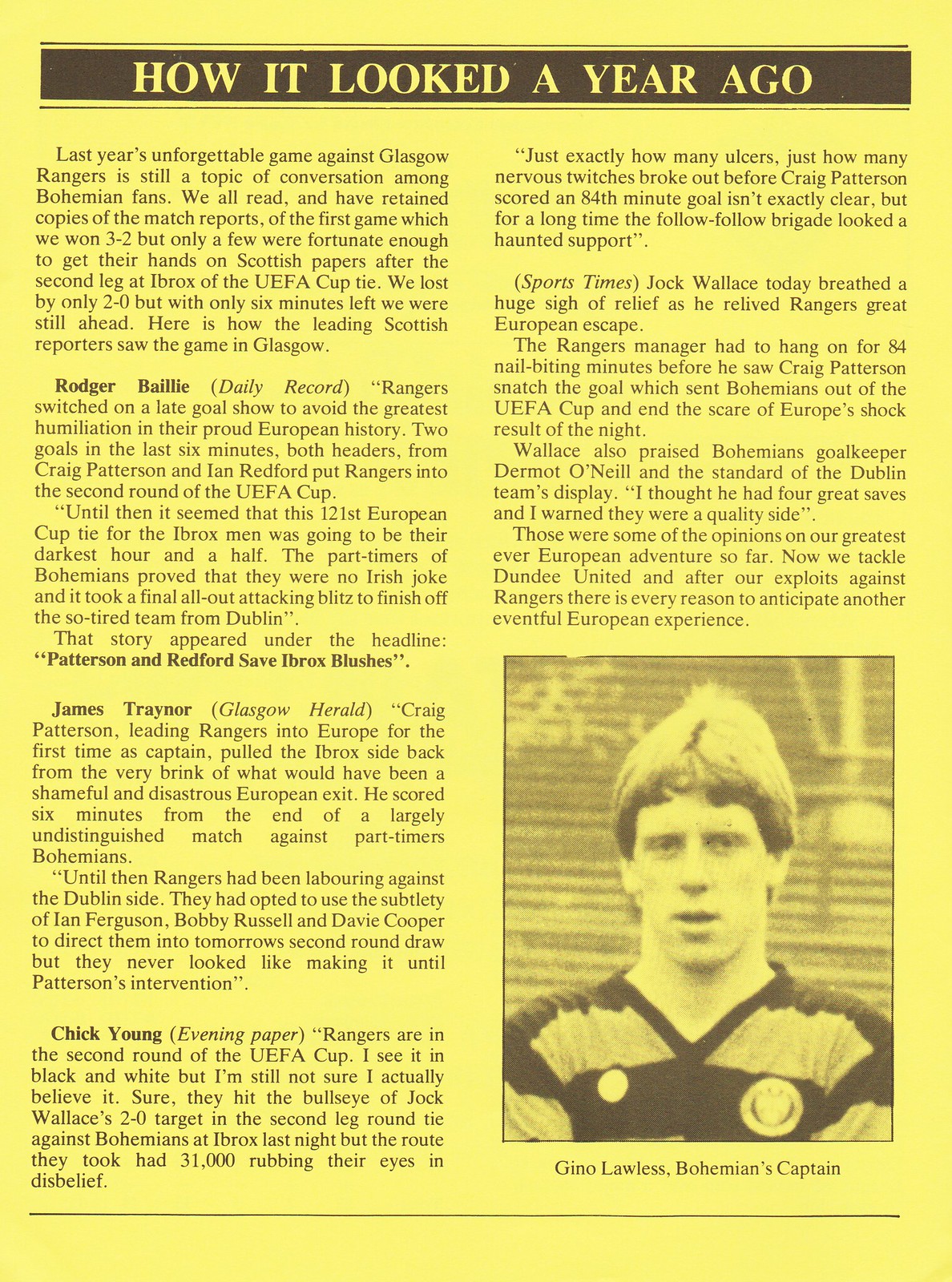This image is a yellow magazine page featuring a detailed two-column spread of black text, topped with a black banner that reads in white font, "How It Looked a Year Ago." The left column begins with the passage, "Last year's unforgettable game against Glasgow Rangers is still a topic of conversation among Bohemian fans. We all read and have retained copies of the match reports of the first game, which we won 3-2, but only a few were fortunate enough to get their hands on Scottish papers after the second leg at Ibrox..." The page discusses the intense matches between Bohemians and Glasgow Rangers, including a 3-2 victory in the first game and a narrow 2-0 loss in the second leg. On the bottom right, there's a gray and black image of Bohemians' captain, Geno Lawless, dressed in a striped V-neck shirt and standing in front of stadium bleachers. The entire page is composed of yellow background with black text, aiming to recount and analyze the memorable football events from a year ago.